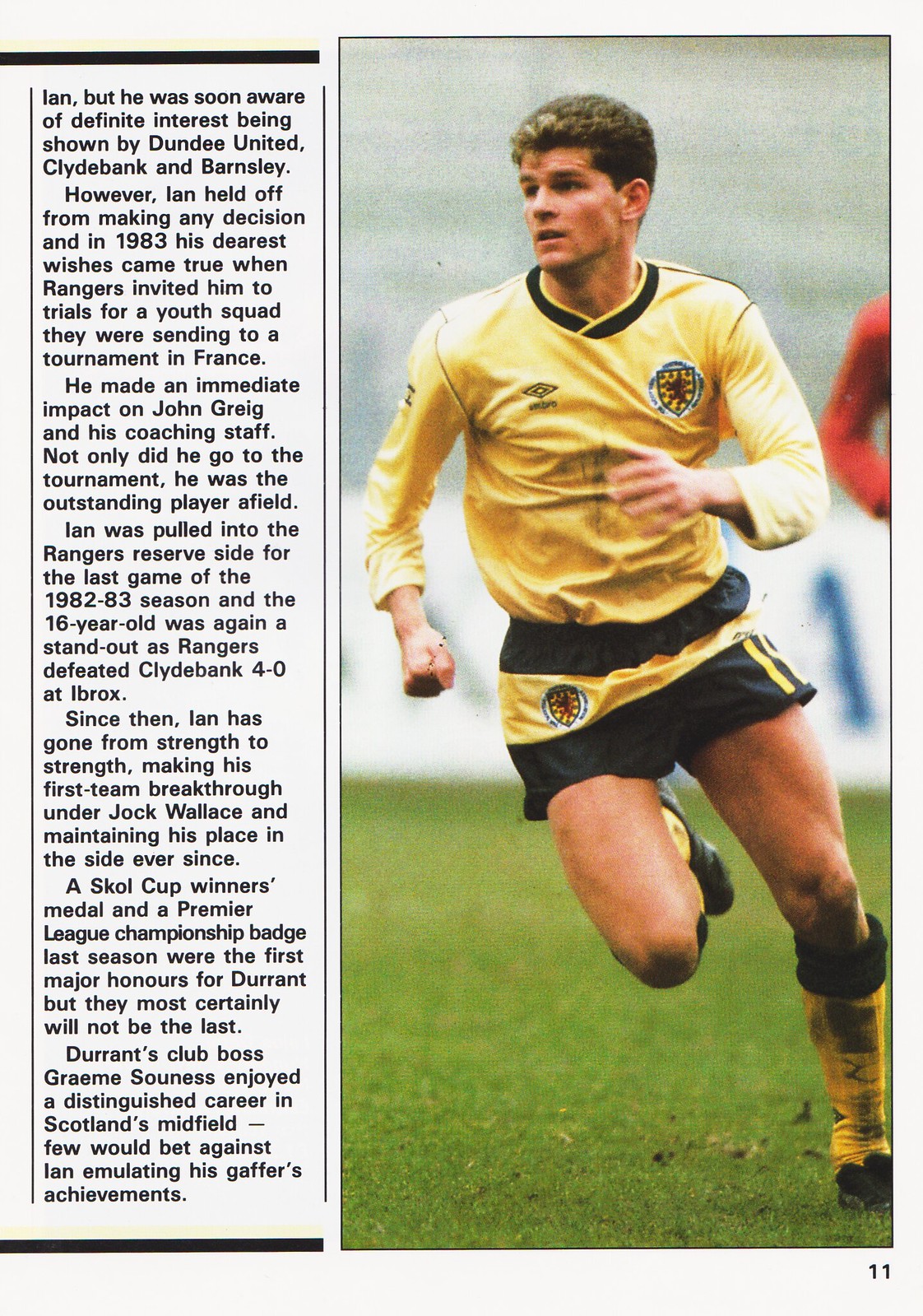The image depicts a page from a magazine or book featuring a soccer player named Ian Durant. The photograph alongside the text shows Ian in action on a grass field, wearing a yellow jersey with black shorts that have a yellow stripe, and yellow and black socks. He has short brown curly hair and appears to be running while making a turn towards the camera.

The accompanying text provides a detailed account of Ian's early career. It mentions that despite interest from clubs like Dundee United, Clydebank, and Barnsley, Ian deferred his decision until 1983 when his dreams materialized with an invitation from Rangers for trials for a youth squad headed to a tournament in France. Making a strong impression on John Greig and his coaching staff, Ian not only participated but was heralded as the standout player. This performance earned him a spot on the Rangers reserve side for the final game of the 1982-83 season, where the 16-year-old shone brightly as Rangers triumphed over Clydebank 4-0 at Ibrox.

Since that pivotal moment, Ian has consistently improved, breaking into the first team under Jock Wallace and securing his position ever since. His dedication and skill have been rewarded with significant honors, including a Skol Cup winner's medal and a Premier League championship badge from the previous season. His current club boss, Graeme Souness, who is highly respected for his own stellar midfield career in Scotland, believes Ian has the potential to emulate his achievements.